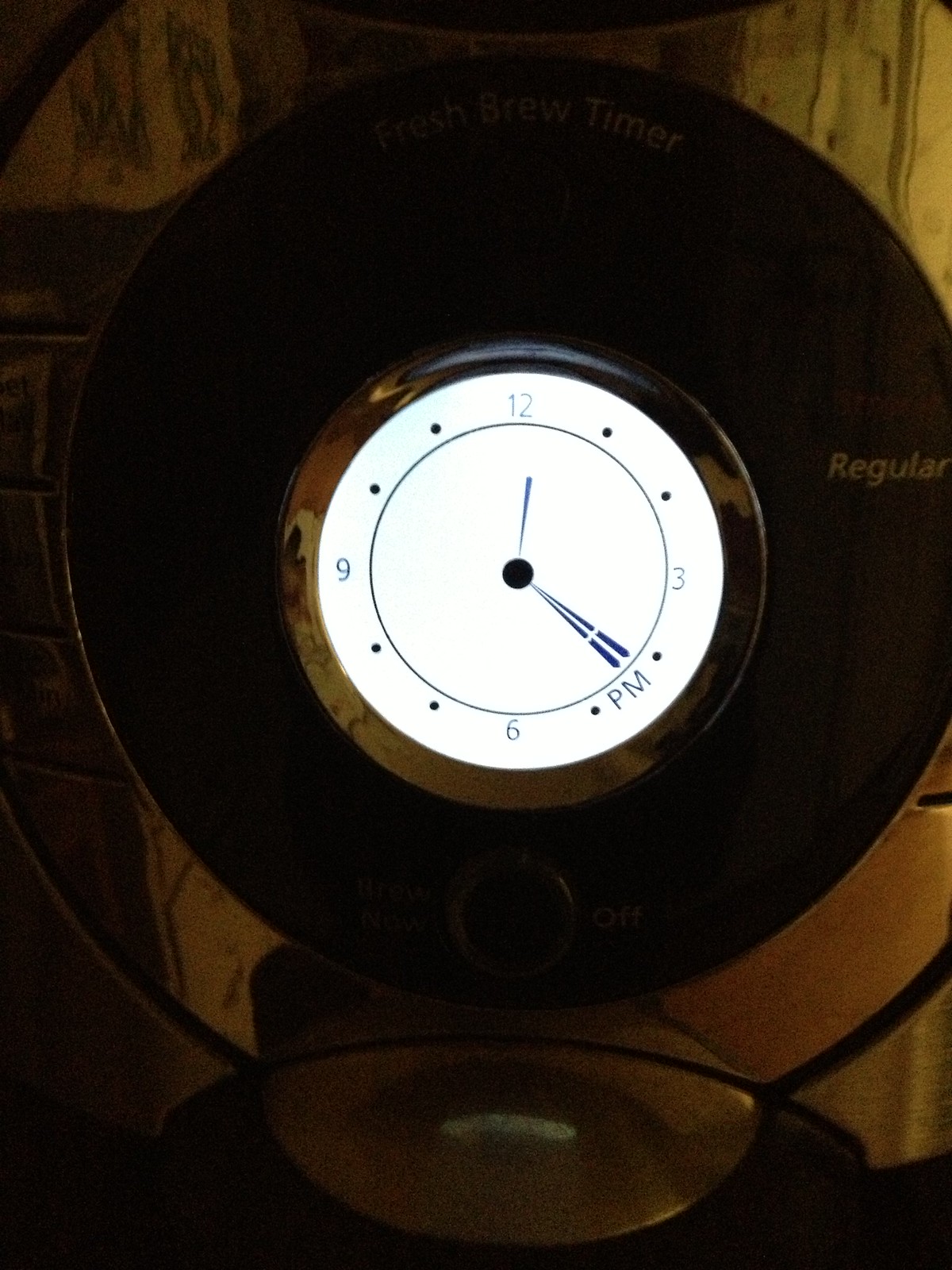This photograph showcases a modern-style clock prominently positioned on a dark-colored table. The background is deliberately blurred, vaguely revealing some horizontal stripes that subtly contrast with the sharp details of the clock. The clock itself features a large, reflective, round frame that draws the viewer's attention. The central area of the clock is distinctly black, reminiscent of a 33 1⁄3 RPM vinyl record, adding a touch of retro elegance.

At the heart of the clock is a silver, round bezel encircling a brightly lit white clock face. The numerals 12, 3, 6, and 9 are clearly marked, with dots signifying the intermediate hours. The clock hands are black and illuminated, converging at a round, black circle at the center of the clock face. The time displayed is 11:20 PM, providing a hint of the serene late-hour atmosphere captured in this image.